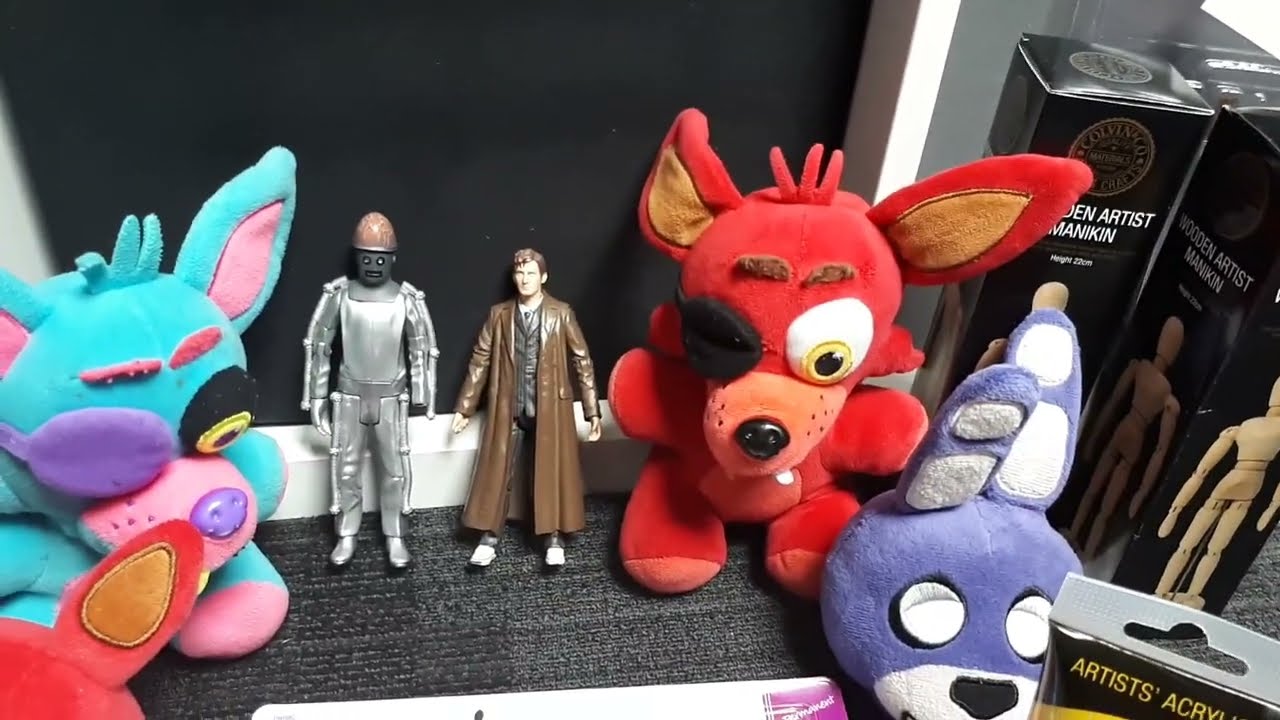The image showcases a detailed and colorful display of stuffed animals and action figures arranged on a gray surface in front of a black background. On the left, there is a turquoise, dog-like stuffed animal featuring a purple eye patch, a black eye with a yellow pupil, a pink nose, and pink accents on its feet and ears. Nearby, a similar red stuffed animal with a black eye patch and tan details on its ears and feet can be seen.

In the center of the image, two distinct action figures are prominently displayed. One figure is dressed in an intricate silver robotic suit with rounded features, including a helmet resembling a brain, round eyes, and a rectangular mouth. The other figure is a man sporting a long, dark brown trench coat almost reaching his feet, a gray vest underneath, brown pants, white shoes, and brown hair.

To the right of these action figures, there's another grouping of items. A stuffed purple rabbit with white eyes and ears is present, along with several black boxes containing miniature artist mannequins used for anatomical reference. Additionally, an "Artist Acrylic" label is visible on one of the boxes, suggesting association with art supplies.